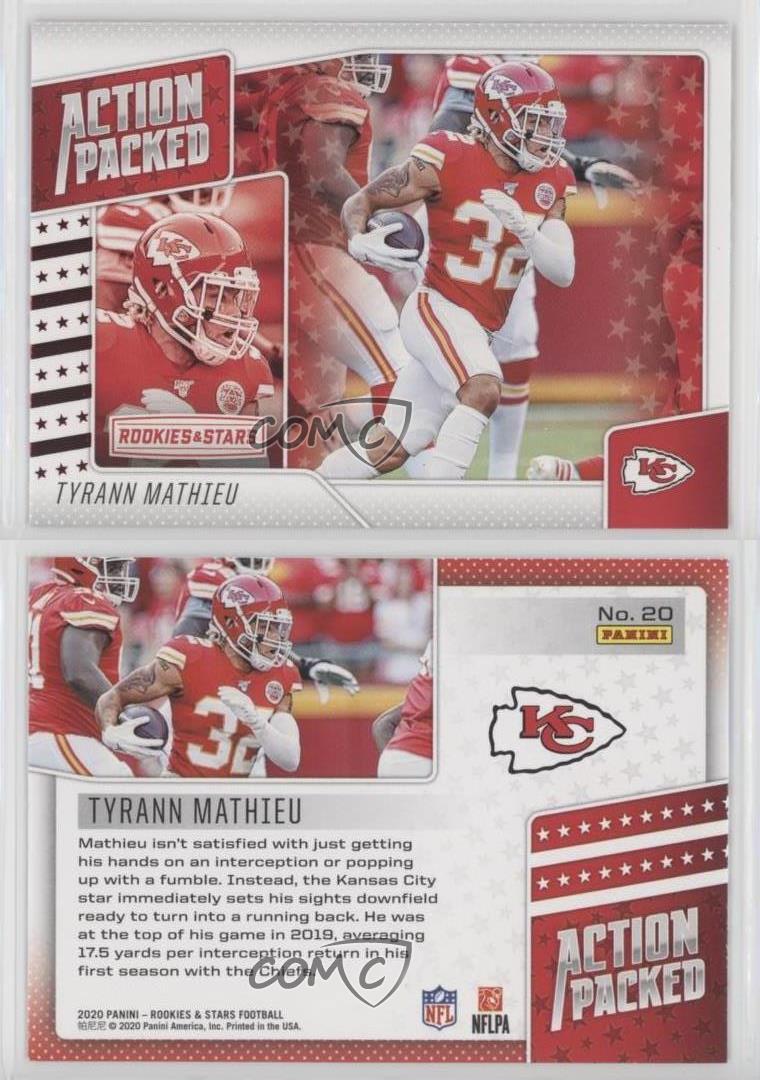This is an image of a 2020 Panini Rookies and Stars football card featuring Tyrann Mathieu of the Kansas City Chiefs. The card is displayed on a screen from COMC and has an indicative watermark at the bottom. The card, titled "Action Packed," shows two clear images of Mathieu. The front features him in action, running with the football tucked under his right arm, wearing a red jersey with number 32, a red helmet, white pants, and white gloves. The background includes other blurred players, emphasizing Mathieu's motion on the field. A close-up of his face is also prominently displayed. The text "ACTION PACKED" is written in all capital letters in white on a red background at the top left of the front image. Below it, Tyrann Mathieu's name is spelled out in capital black letters. On the back of the card, the same image of Mathieu appears along with a brief description indicating his relentless approach to the game, noting his eagerness to not just intercept passes or recover fumbles, but also turn plays into significant advances downfield. The card is numbered 20, visible at the top right above the Panini logo.